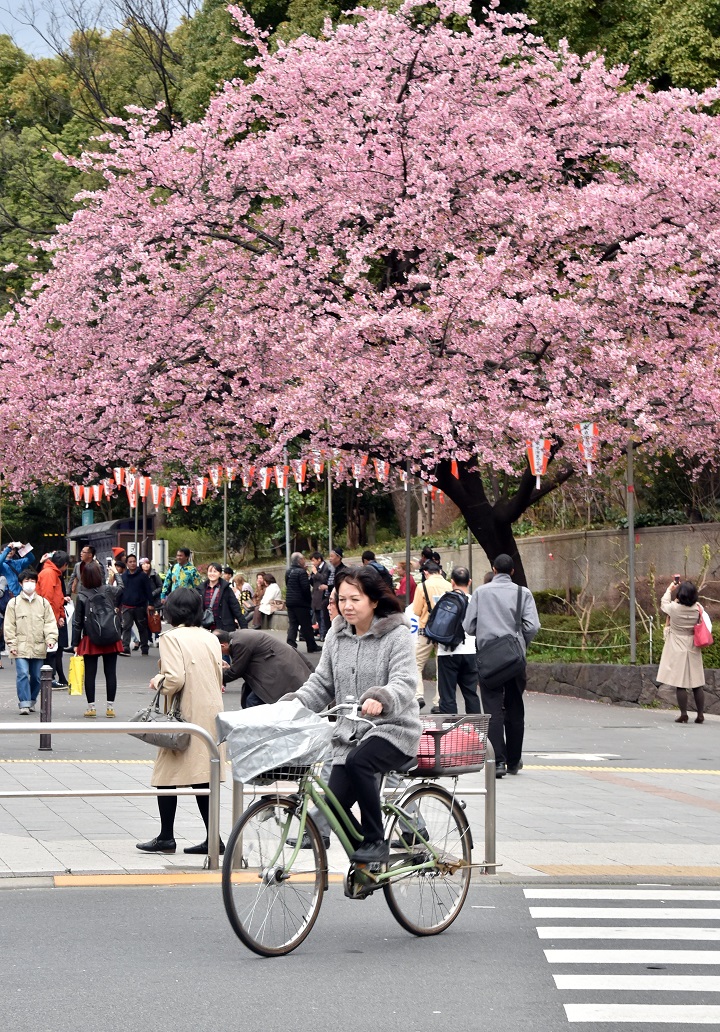In this vibrant image, we see a bustling scene centered on a woman riding a green bicycle along a crowded asphalt walkway. The woman, with shoulder-length black hair, is dressed in a gray jacket with a fur-lined hood and matching cuffs. She steers her bike, which features a black wire basket at both the front and the back—carrying a gray bag in the front basket and a pink bag in the rear basket. The walkway is teeming with people, drawing attention to a large, striking cherry blossom tree in full bloom, adorned with beautiful pink and orange flowers. The tree dominates the background, under which a woman in a white coat stands on a sidewalk, capturing a photo of the vibrant blossoms. This picturesque scene is further enhanced by small lanterns hanging beneath the tree, contributing to the festive atmosphere. To the left of the cyclist, several more pedestrians, including men with backpacks or cameras, add to the lively urban tableau, all seemingly captivated by the magnificent cherry blossoms above.